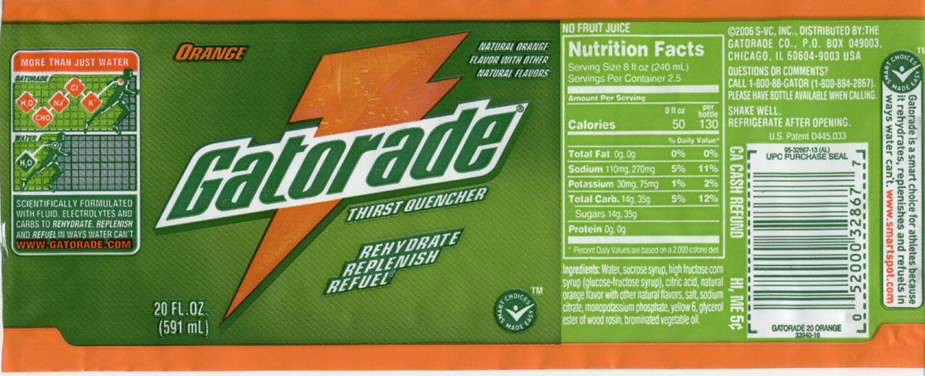This photograph showcases a flattened Gatorade label, featuring a vivid and detailed design. The label is rectangular, bordered by orange strips at both the top and bottom edges, giving it a distinctive frame. The main background is a striking green, with a gradient effect transitioning from darker to lighter shades on the left-hand side.

On the left side of the label, there is a white-outlined rectangular box with multiple sections. The top section includes an orange strip, followed by three smaller rectangles within. The upper two rectangles have a grid pattern and depict a filled-in silhouette of a person walking, viewed from the side. 

Dominating the center of the label is the iconic Gatorade logo, characterized by a bold orange lightning bolt. The word "Gatorade" is displayed prominently in green letters, set against a white background that stretches horizontally across the lightning bolt.

The right side of the label presents a lighter green color, which is actually the back of the label. It contains the nutrition facts box on the left side, filled with white text detailing the product's nutritional information. Above the nutrition box, there is additional white text, and below, there's a white rectangular UPC code. The UPC code includes green lines and numbers, completing the detailed and informative design of the Gatorade label.